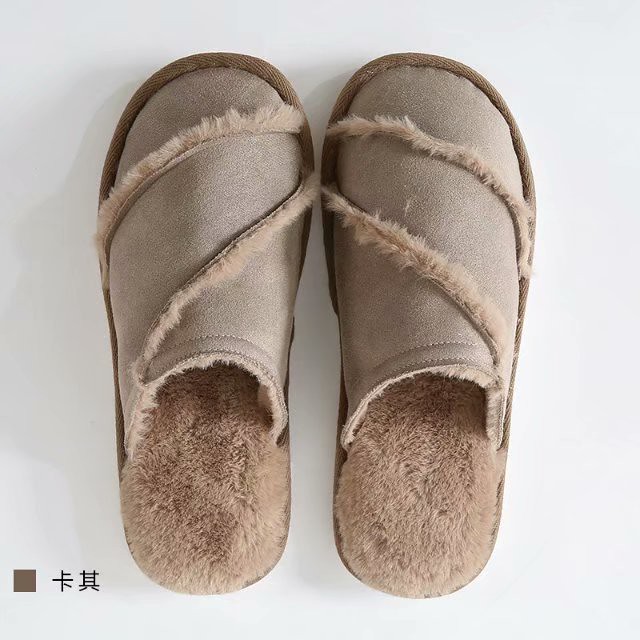This image displays a close-up of a plush pair of men's slippers set against a plain white background. The slippers are a light coffee brown or taupe tan color, featuring a luxurious fur lining on the inside and a soft, plushy texture that mirrors a carpet. The exterior appears to be made of a leathery material, sewn together in a pattern where the seams, adorned with the same fluffy fur, create a graceful curve around the tip and central part of each slipper. The lining seamlessly matches the fur on the inside, enhancing comfort and consistency in design. Additionally, in the bottom left corner of the image, there is a small brown square next to two black kanji characters, suggesting a possible Chinese or Japanese origin or inspiration.